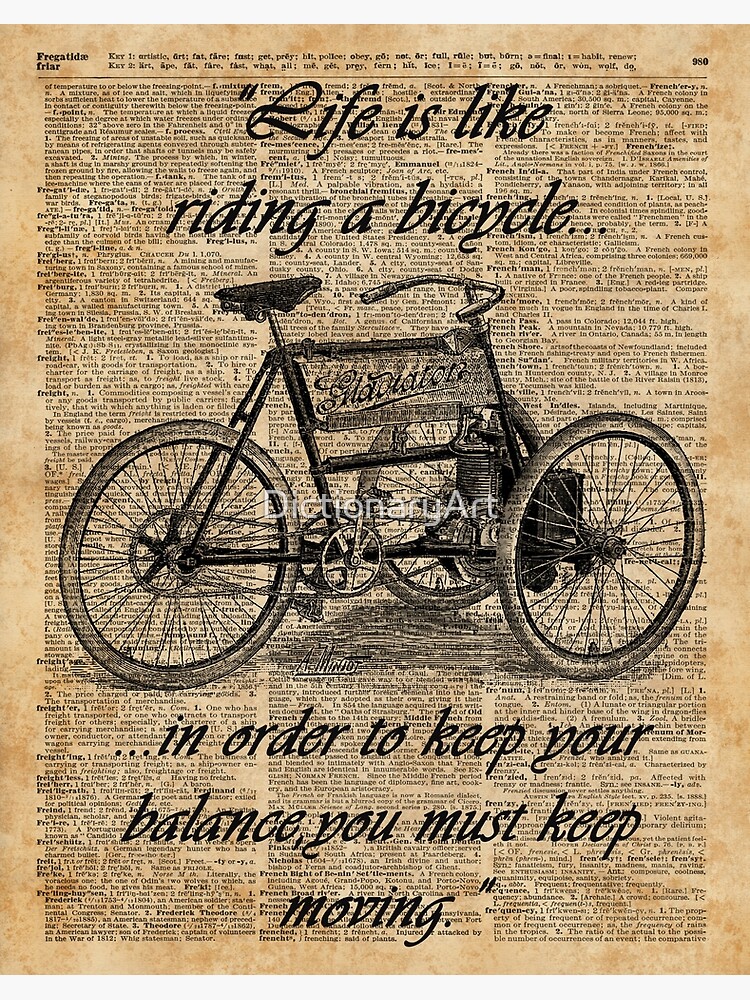This detailed description merges insights from three different observations:

The image is of a vintage, tea-stained dictionary page, yellowed with time and featuring darker tan blotches. The page is from a dictionary and includes definitions of words starting with F, specifically from "Fregatide" to "Frequency." Located at the top left of the page are the words "Fregatide" and "Friar" in black print, while "Frequency" is at the top right, accompanied by the number 980. Between these words are lines that read "Key 1" and "Key 2," with corresponding words and accent marks. 

Superimposed on this aged page is an ornate black cursive script that reads, "Life is like riding a bicycle...". Below this quote is a detailed black and white illustration of a vintage tricycle—distinguished by its two wheels at the back and one at the front—with a leather seat and a handlebar. Below the tricycle illustration, the quote continues in black script: "...In order to keep your balance, you must keep moving." There is also a watermark in white at the bottom of the image, branding it as "Dictionary Art."

Overall, the composition combines the antique aesthetic of the dictionary page with an inspirational quote and a vintage tricycle illustration, creating a nostalgic and motivational piece of art.